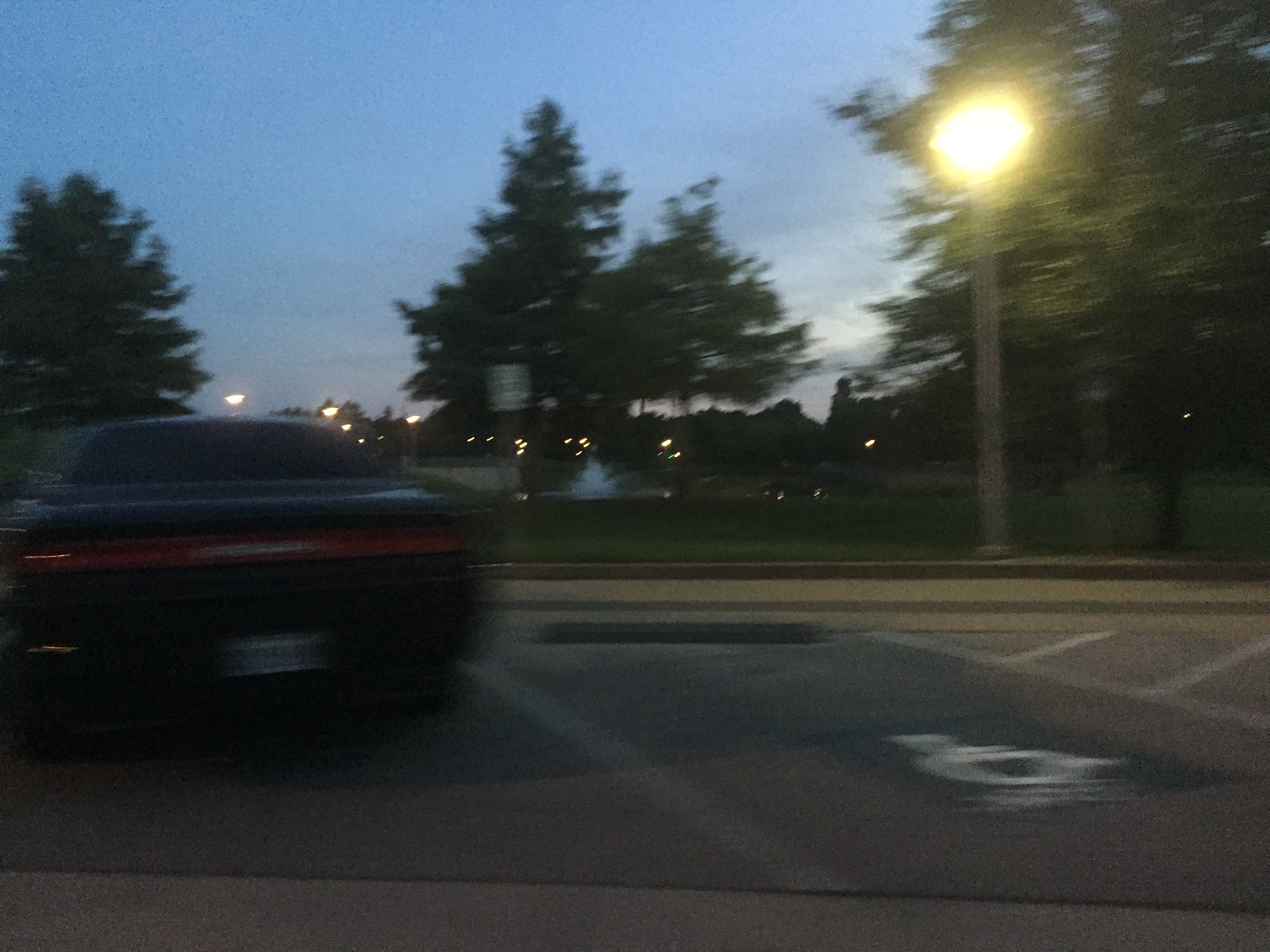In this photograph taken at dusk, the scene is set in a dimly lit parking lot. The sky overhead remains a twilight blue, transitioning to darker gray hues that signal the impending sunset. Wisps of white and light blue clouds hover near the horizon. 

Dominating the left side of the image is a dark-colored sedan, possibly black or dark blue, parked next to an empty handicap parking spot. The sedan features elongated rectangular red taillights and a blurred license plate. The handicap spot is clearly marked with a white logo and bordered by white lines; on the right side of the spot, diagonal lines indicate an area where parking is not allowed. There's a rectangular stanchion, likely intended to prevent vehicles from driving too far forward.

To the right of the sedan, a yellow-glowing streetlamp rises from a dark gray cylindrical post, casting a warm light that combines white and orange tones. The light illuminates a portion of the parking lot, contributing to the overall nocturnal ambiance of the scene. 

In the background, additional streetlights can be seen, faintly glowing as night approaches. A silhouette of trees spans the horizon, varying from dark green to slightly lighter hues closer to the streetlamp, enhancing the depth of the landscape. The photograph, although slightly blurry, captures the tranquil, transitional beauty of early evening with subtle yet intricate details of the surroundings.